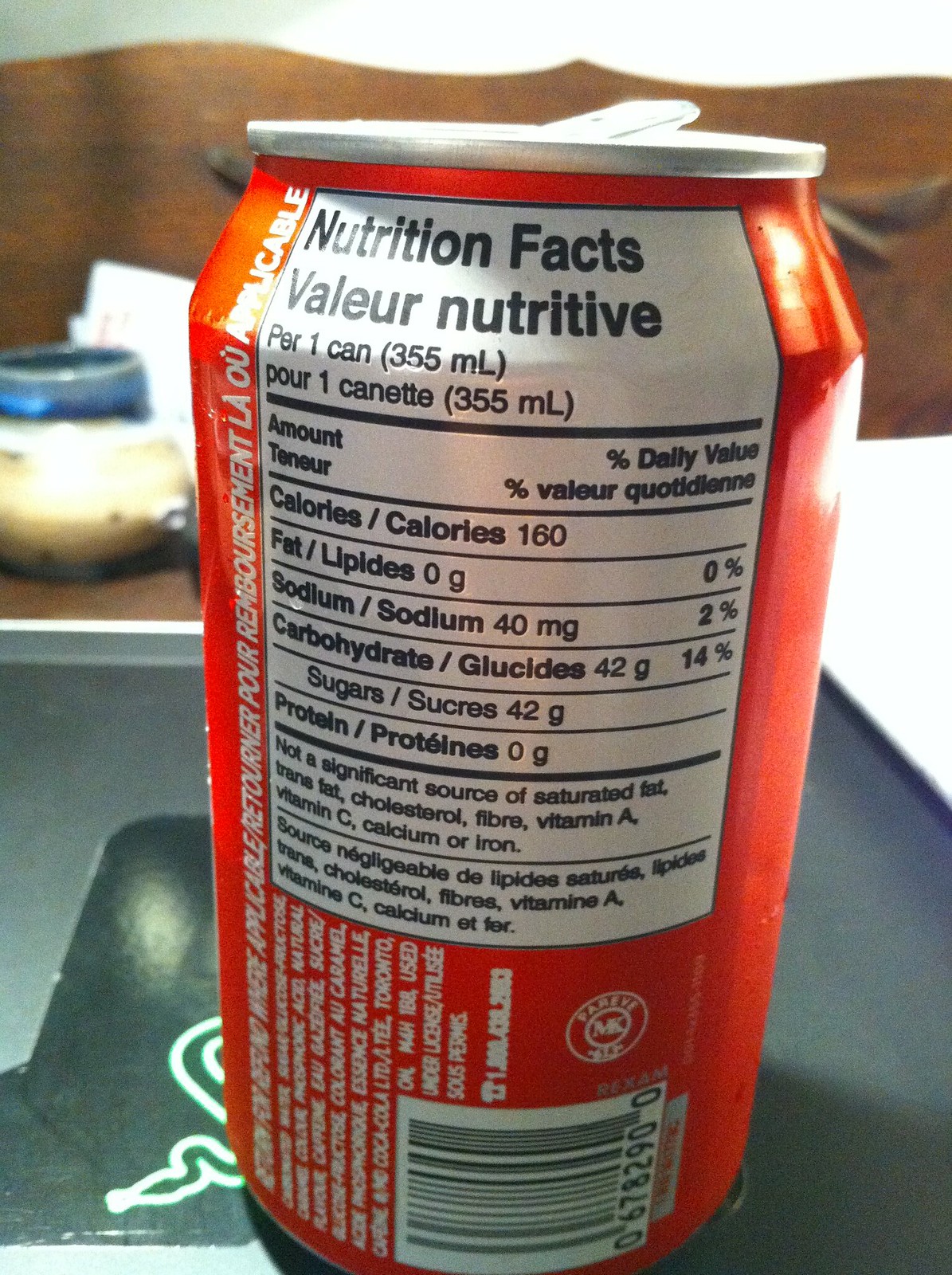This color photograph showcases the back of a silver drink can, prominently featuring a large nutritional facts label that occupies more than half of the can's surface. The label, written in black text, provides detailed information including serving size, nutritional values per one can, and various readings for calories, fat, sodium, carbohydrates, and protein, among others. The can has a distinctive reddish band encircling its lower portion, which bears sideways text that is somewhat difficult to decipher. At the very bottom of the can, there is a barcode presented in black on a white background.

The can is situated on a black tray. To the left of the can's base, there is an intriguing design resembling a pair of darker black boxing gloves adorned with a white cord and black lining. In the background, a wooden surface extends horizontally, topped by a grey or white wall. To the left side of the image, a white jar with a blue round lid can be seen alongside another white object. Just to the right of the can, there appears to be a white, squarish object adding to the composition of the scene.